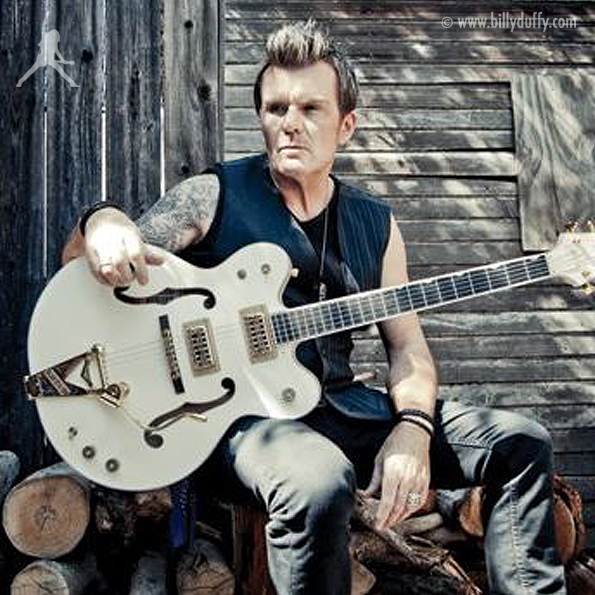In this slightly low-resolution photograph, a white male is seated in front of a building with wood siding that evokes a farmhouse or cabin aesthetic. Centered in the image, he looks off to his right, towards the left of the frame. His hair, styled in a gelled, rock-star look, complements his tank top and dark jeans. On his right arm, he sports a full sleeve of tattoos. He holds a large electric-acoustic guitar, predominantly white with metallic accents and black details, across his lap with his right hand, while his left hand rests on his knee. Adorning his neck is a necklace with an emblem, accompanied by a ring and bracelets on his hands. Beside him on the ground are chopped logs of wood. The top left corner of the photograph features a logo of a person playing an air guitar, while the top right corner displays the text "www.billyduffy.com." The image, rich in details such as brown, white, black, blue, and gray hues, appears to be taken professionally.